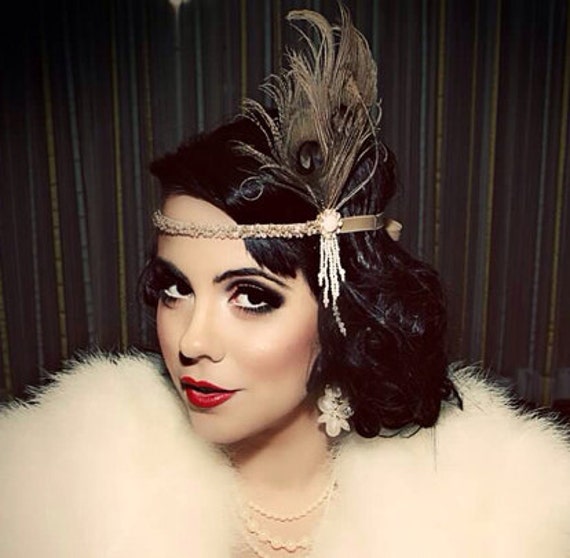The photograph features a woman dressed in a 1920s flapper-inspired costume. The image is a close-up shot from the head to the shoulders, showcasing her detailed attire and makeup. She has short, slightly curly dark hair and is adorned with a headband that includes bundled peacock feathers and intricate beaded detailing. Her makeup is pronounced, featuring dark eyeshadow, heavy lashes, thin black eyebrows, bright red lipstick, and noticeable blush on her pale cheeks. She is wearing a white marabou feather coat or shawl with three strands of pearl necklaces, and an ornate, large earring peeks out from her hair. The background consists of vertically striped fabric in green, blue, and possibly other colors. She is looking directly at the camera, exuding an aura of nostalgia and elegance characteristic of the Roaring Twenties.